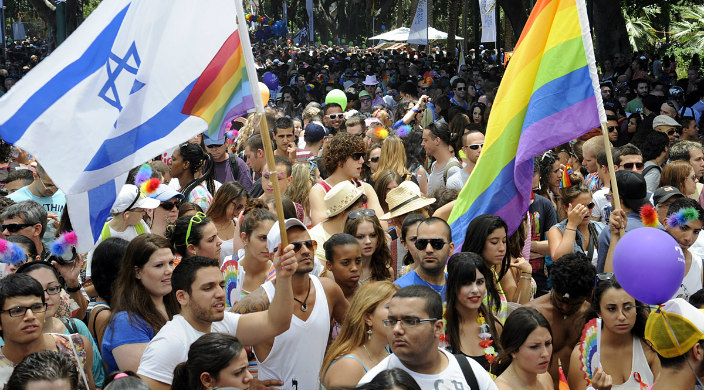The vivid photograph captures a bustling scene, likely from a pride parade or demonstration, teeming with a diverse crowd of people. Dominating the image are vibrant colors, with numerous figures brandishing large and small rainbow flags, indicative of LGBTQ pride. Prominently, a large Israeli flag, characterized by white and blue stripes and a central Star of David, is held high by a person in a white t-shirt. Attached to this Israeli flag is a smaller rainbow flag, signifying inclusivity.

The crowd is tightly packed, suggesting thousands of attendees. Many individuals, dressed in summer attire of tank tops and t-shirts, are donning sunglasses, hats, or visors to shield themselves from the apparent heat. In the lower right corner, a purple balloon stands out, along with a woman in a white tank top holding an open rainbow fan. Additionally, scattered throughout the throng are colorful balloons—including green, blue, and yellow—enhancing the festive atmosphere.

The background hints at the setting being outdoors with visible trees, possibly along a parade route or in a park, and there are indistinct signs and possibly tents in the distance. The crowd, mostly young and diverse, conveys a spirited yet peaceful gathering, unified in its celebration or cause.